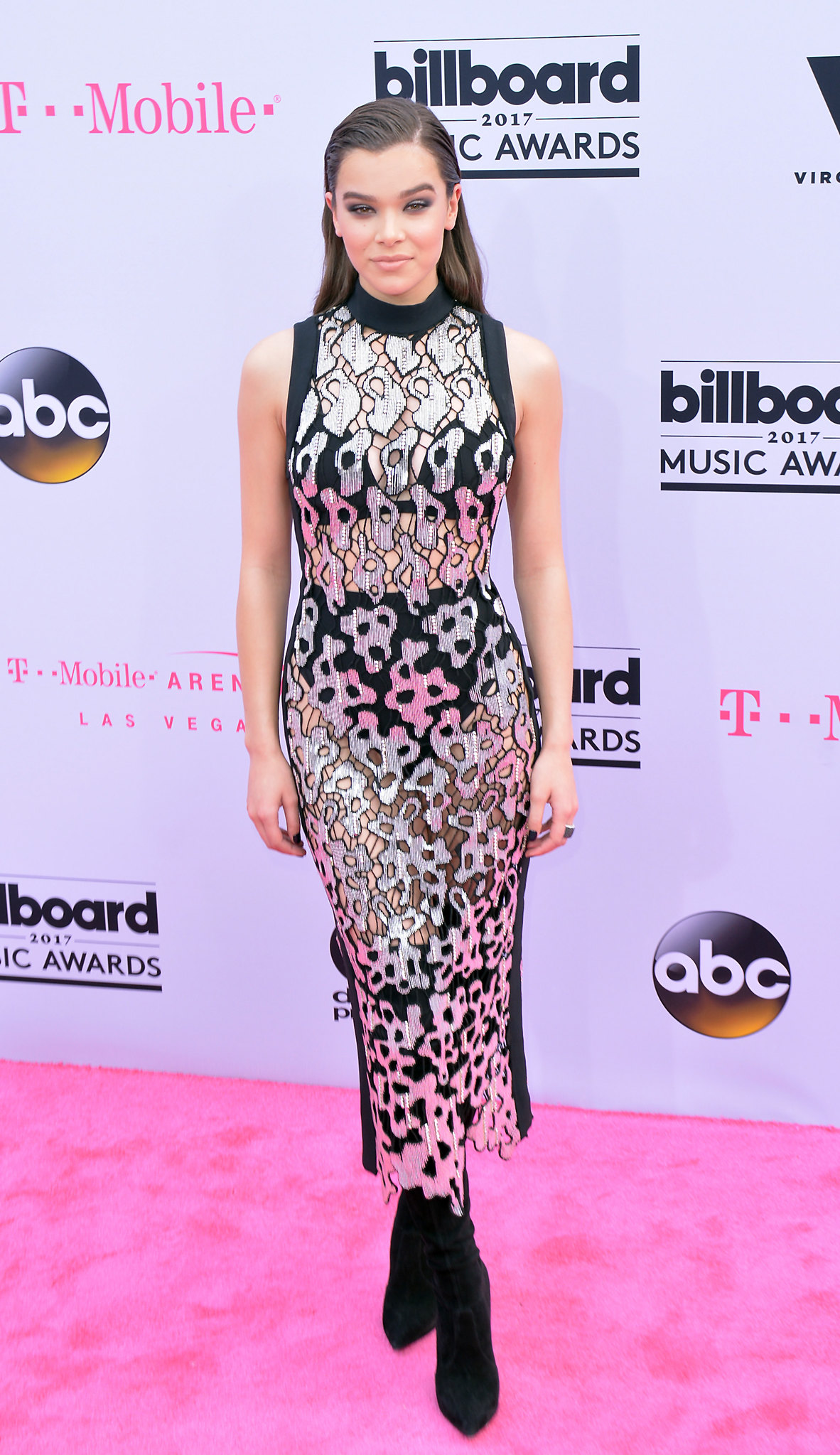In this image, we see a young white actress posing at the 2017 Billboard Music Awards. Behind her is a lavender backdrop adorned with logos from T-Mobile, ABC, and the event itself, all repeatedly patterned across the board. She stands confidently on a bright pink carpet with her legs slightly crossed and her arms at her sides, gazing directly at the camera.

Her straight, dark brown hair is slicked back and cascades down to the middle of her back. She wears a striking strapless gown that merges elegance with a hint of edginess; the dress features a black collar and black edging around the sleeveless sections. The gown itself comprises a shimmering silver fabric interspersed with what resembles intricate, transparent splotches, creating an almost painterly effect. Adding to its uniqueness, the dress contains subtle hints of gold around the waistline, only partially visible beneath the silver overlay, giving the appearance of a hidden golden waistband.

Her footwear adds to the ensemble’s boldness, with black boots or shoes peeking from beneath the gown. She also sports makeup that accentuates her features, completing her glamorous look for the evening.